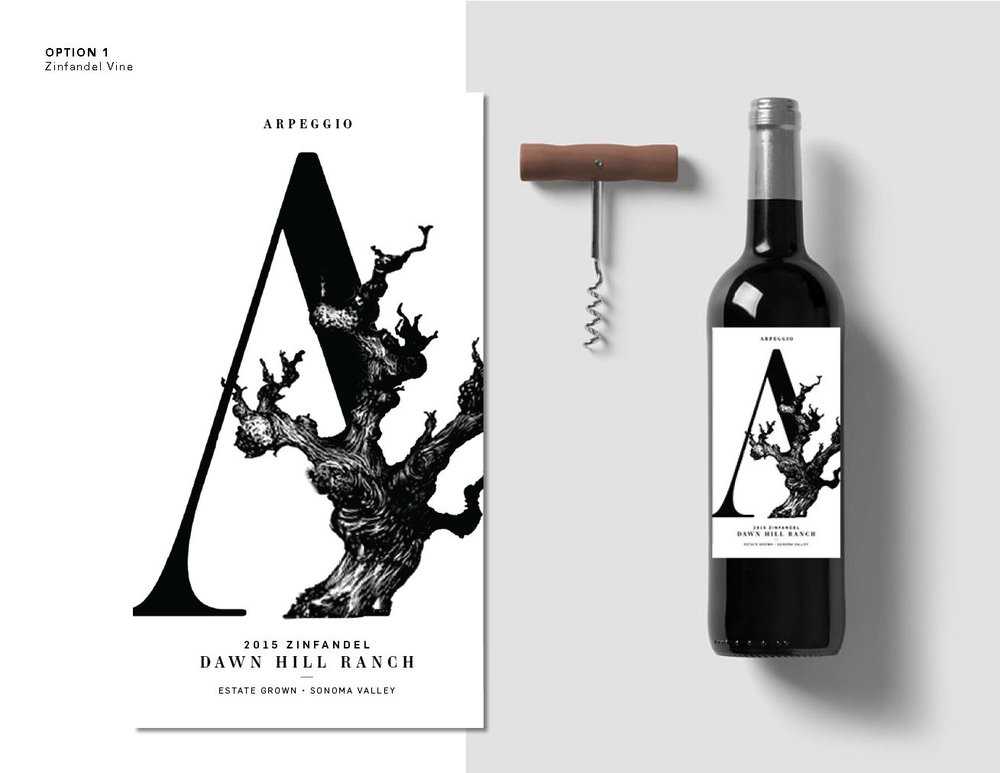The photograph features a professional advertisement for Arpeggio wine, specifically highlighting their 2015 Zinfandel from Dawn Hill Ranch, estate grown in Sonoma Valley. The image is set against a pristine white background, drawing attention to the intricacies of the wine's branding. Dominating the left side is a detailed close-up of the wine label: a large, stylized letter "A" formed with a gnarled tree trunk and branches. Above this letter, "Arpeggio" is delicately inscribed, while below, the wine's vintage and origin are clearly stated. To the right stands the actual wine bottle, dark and elegant, adorned with the corresponding white label and silver foil around the cork. Beside the bottle rests a corkscrew, featuring a brown handle and silver bottom, completing the sophisticated and inviting presentation of the product.